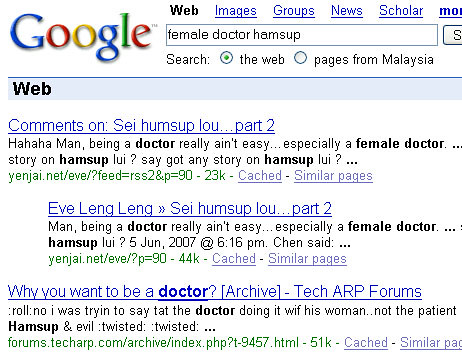The image is a screenshot of an old Google search page. Positioned centrally, the screenshot captures the classic, multicolored Google logo at the top left, with letters in blue, red, yellow, green, and red. At the top, there are navigation links for "web," "images," "groups," "news," and "scholar," indicating that the "web" tab is currently selected. The search query in the field reads "Female Dr. Hensup," and the search appears to have been executed. An option for searching "pages from Malaysia" is visible but unchecked. The search results display three links, though the exact websites are blurry. The legible portion of the last result reads, "Why you want to be a doctor, archive, tech, ARP forums." The overall aesthetic suggests the screenshot may be from an older version of Google, possibly from around a decade ago.